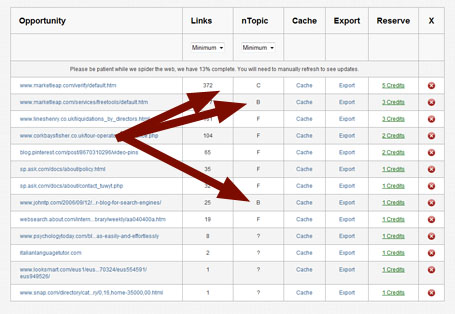This image depicts a detailed graph related to "Opportunity," prominently indicated in the upper vertical column. The graph features various sections labeled as "Links," "Topic," "Cash," "Reserve," "Export," and "Reserve." Below these labels, the text reads, "Please be patient," accompanied by numerous small, illegible words.

The layout includes categories highlighted in blue and three maroon arrows originating from a single blue category. Two of these arrows point towards "Links" and "Topic," while the third also directs to an endpoint labeled "Topic." Under the "Reserve" section, the graph emphasizes green text specifying the number of credits available. Adjacent to this section is an "X" column, characterized by red circles with X's inside each.

Despite its detailed structure, the graph lacks an explicit explanation of its content, providing no further context beyond the overarching label of "Opportunity" in the subject column on the left side.